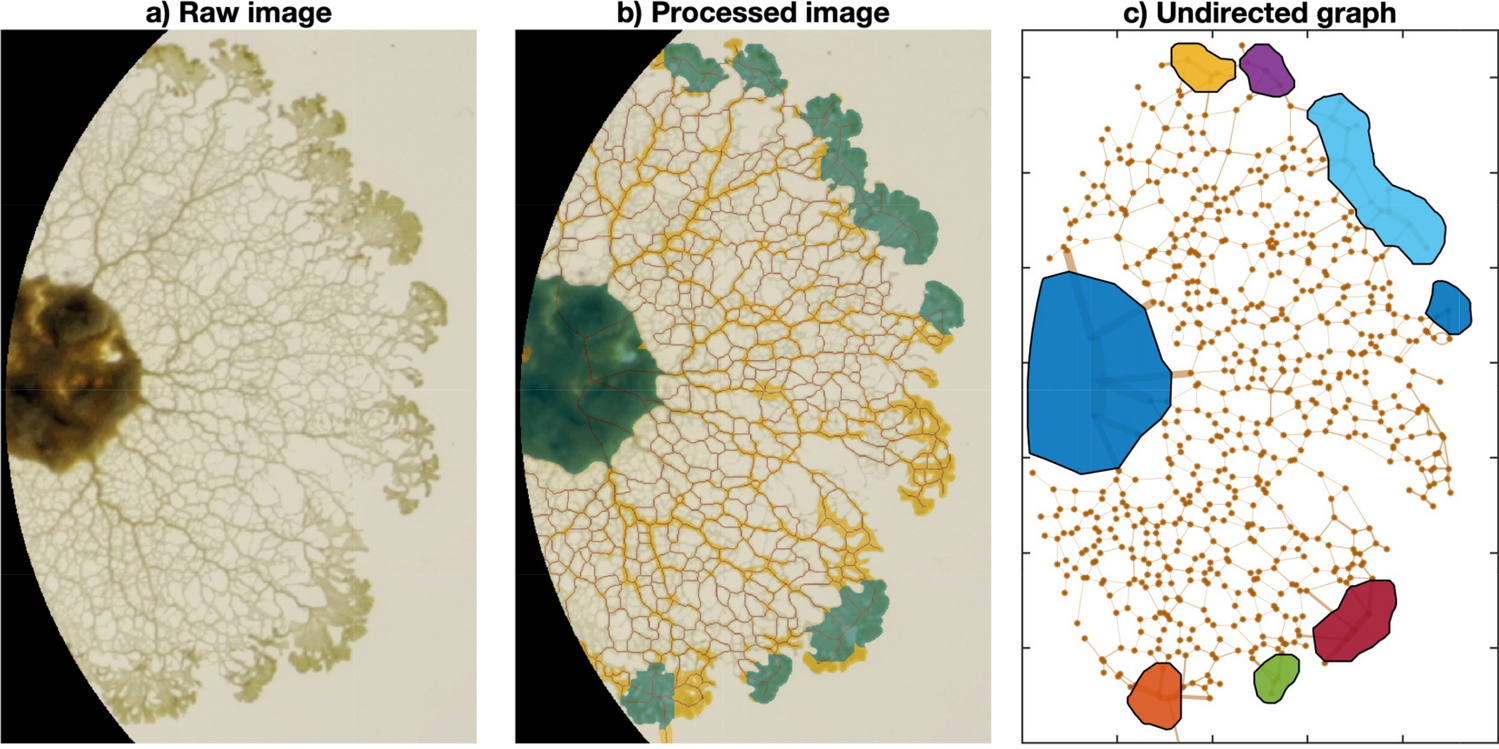The three-panel image sequence, likely from a scientific textbook, illustrates the transformation of a raw visual data sample into a processed form and subsequently into a graphical representation. Panel A, labeled "raw image," exhibits a partially visible circular shape on a black background, featuring a gold-colored, irregular blob at its center. This central blob is encircled by a delicate network of ink-like extensions resembling a barren tree's branches. 

Panel B, titled "processed image," retains the original structure but alters the coloration. The central blob shifts to a turquoise hue, with additional turquoise splotches appearing at the outer edges of the network. The intricate web of branches intensifies in color to a darker yellow.

In the final Panel C, "undirected graph," the central blob is rendered as a blue outline. The previously gold branches are replaced by an interconnected network of orange-brown lines, terminating in variously colored dots and nodes. These nodes include a variety of colors such as yellow, purple, blue, red, and green, dispersed across the image. This panel abstracts the initial structure into a simplified graphical format, highlighting the connectivity of the network.